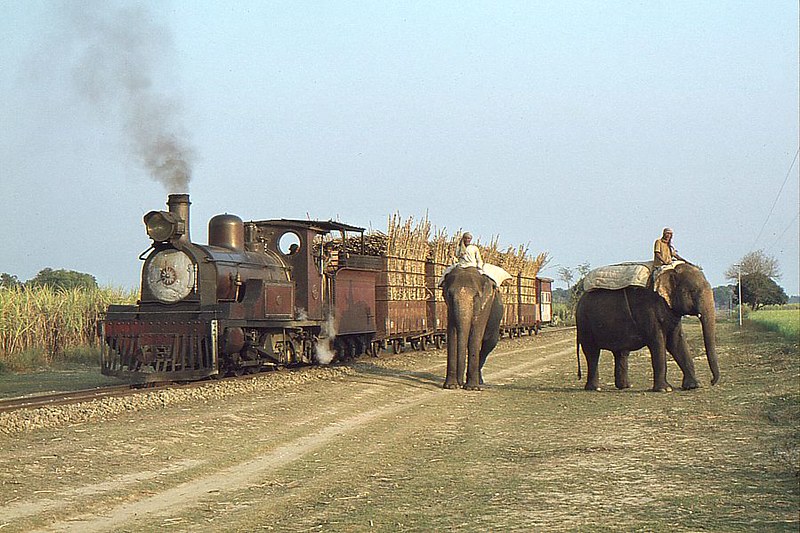The image depicts a rustic country scene, likely set in India. A dirt road winds through the landscape, flanked by a narrow gauge train track. The focus of the scene is a small, antique steam engine, which is chugging along with a couple of cars in tow, laden with harvested hay or grain. Smoke billows from the train’s chimney and engine compartment, adding to the nostalgia of the moment. To the side, amidst parched grass and some sparse trees, stand two elephants draped with blankets. Perched on the elephants' necks, two men dressed in robes and tunics ride with a calm dignity. In the background, a cornfield stretches out, completing this picturesque tableau of bucolic life.